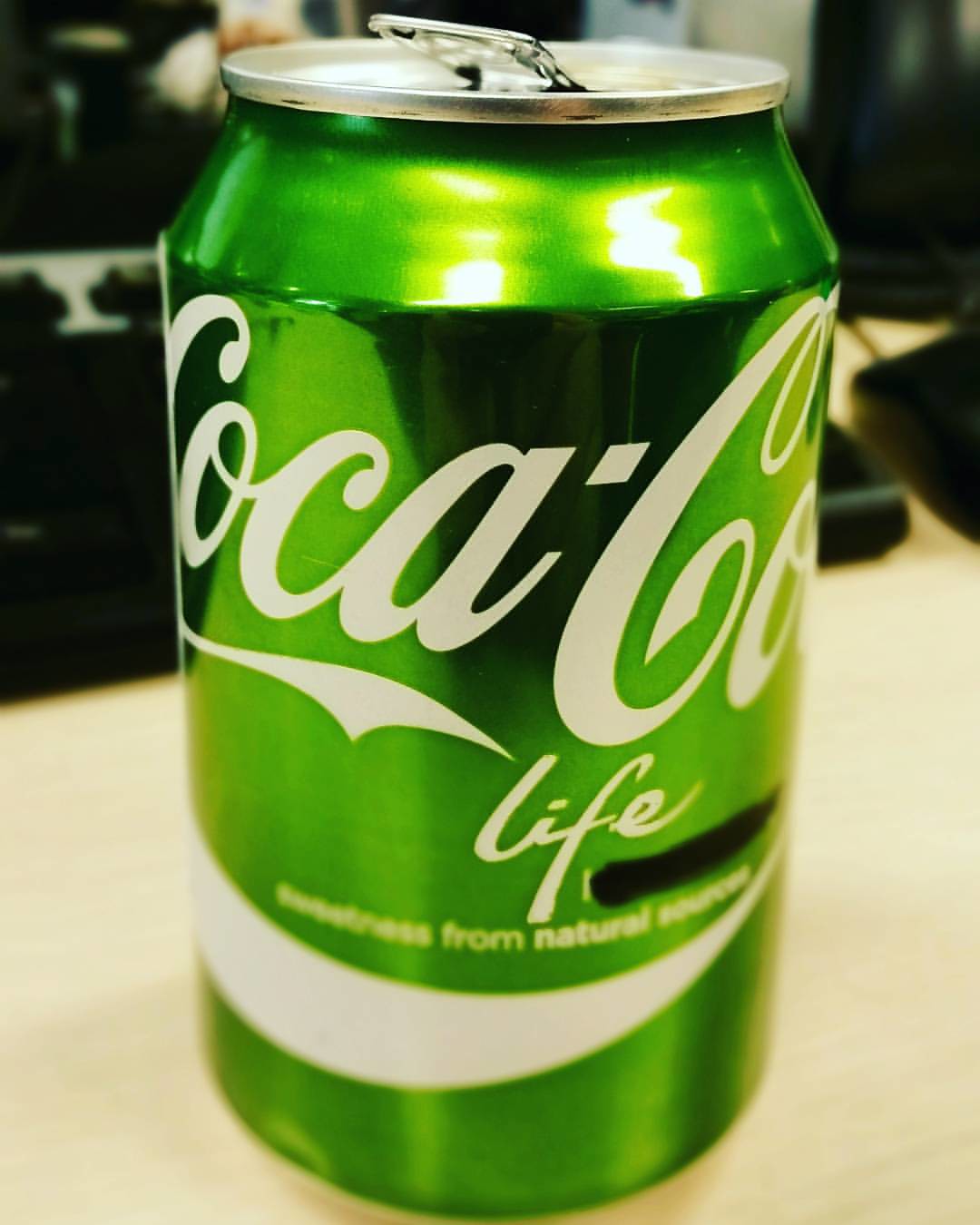This close-up photograph features a shiny, apple green Coca-Cola Life can with white lettering. The can, prominently displayed and in focus, sits atop a blonde-colored wooden table, while the background is out of focus, revealing some indistinct black rectangular objects and light and dark areas. The Coca-Cola Life logo is written in typical Coca-Cola script, with "Life" in a calligraphy-style font. Below the logo, it says "sweetness from natural sources." The can has an open, metallic aluminum tab and a black mark near the bottom. There are reflective lights visible on the top of the can, highlighting its glossy finish.